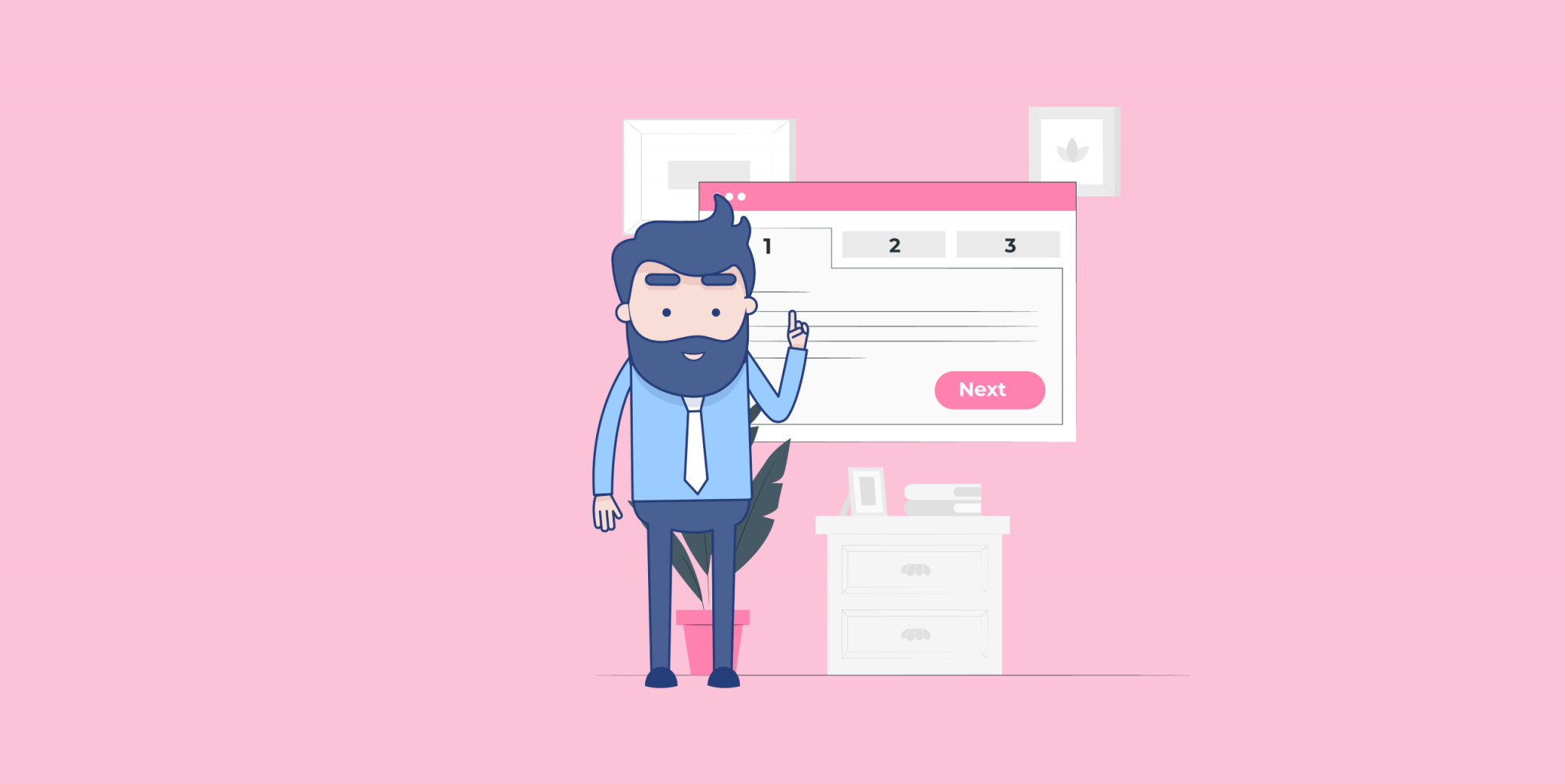The image features a simplified cartoony scene set against a completely pink background. At its center stands a man with wavy gray hair, gray eyebrows, and a full beard and mustache, rendered in a light-hearted and minimalist style. He is wearing a light blue dress shirt, a white tie, black pants, and black or dark-colored shoes. His right arm points downward while his left arm points up towards a floating computer-like window with three tabs labeled 1, 2, and 3, and a prominent pink 'Next' button.

Behind the man is a potted plant with a pink base and green foliage. To the right of the plant, there is a white cabinet adorned with a picture frame and a couple of books. Above this cabinet floats another screen-like element featuring lines of text and a small image of a leaf to the left, further contributing to the tutorial or instructional theme of the image. The overall color scheme prominently features shades of pink, baby blue, and white, blending harmoniously to create an eye-catching and instructional visual.